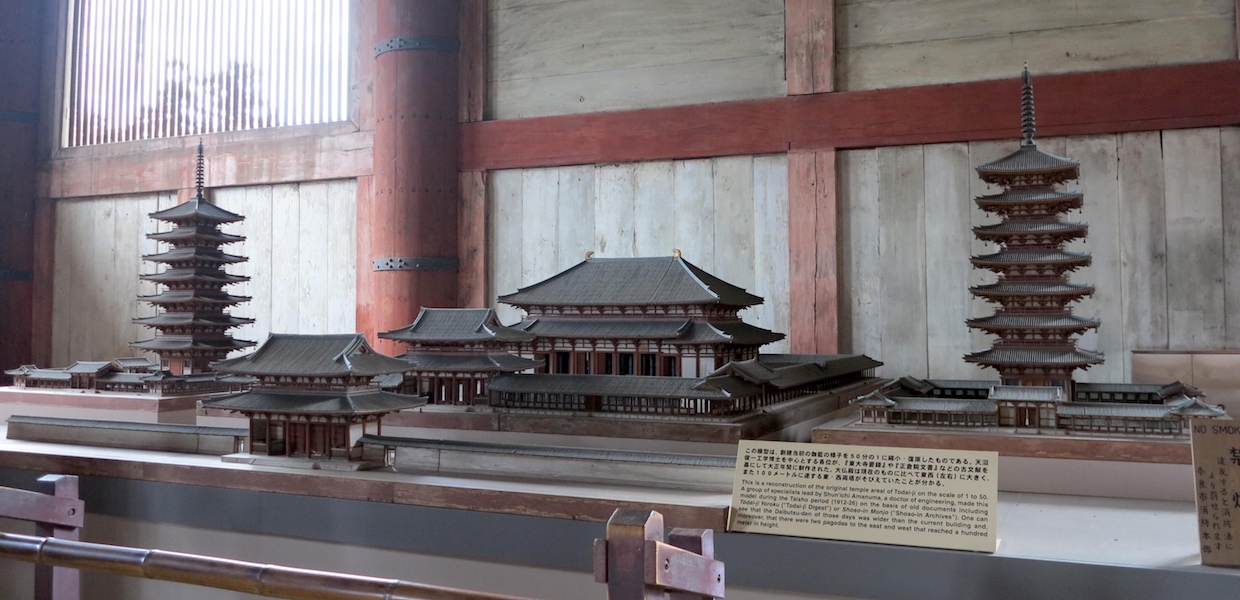The image showcases a detailed miniature model of traditional Japanese temples, meticulously styled and crafted from reddish-brown wood. Positioned on a long shelf or table, this architectural design is intended for engineering and architectural purposes, providing a scaled-down preview of what the actual structures will look like once built. The scene includes several Asian-style buildings arranged with a central focus; a larger but shorter building with a pagoda-style roof is flanked by tall towers on either side, each adorned with antenna-like structures at their peaks. In front of the display, an informational plaque written in Kanji provides context and description of the model. The background features a mix of wood panels, rust-colored beams, and light gray concrete walls, with one panel incorporating a clear window. The photograph, captured indoors, displays dark and muted colors, enhancing the serene and traditional aesthetic of the miniature temples.